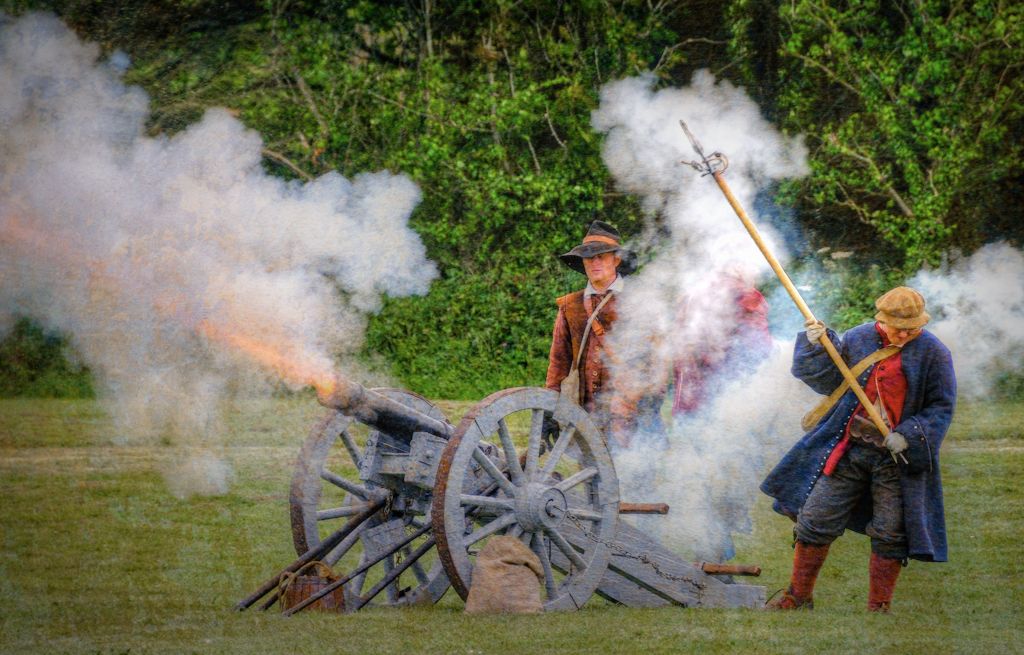This image captures a vivid scene of a historical war reenactment, featuring a cannon mid-fire with flames and thick smoke billowing from its gray barrel. The cannon, which has two large wooden wheels, rests on a grassy field. In the foreground to the right, one person dressed in 17th or 18th-century attire is holding a long igniting rod. This individual wears a blue poncho-like jacket over a red shirt, dark pants, red knee-high socks, and a tan hat. Nearby, another person is seen in a brown vest, rusty red undershirt, and a black wide-brimmed hat with a tan band. The background is lush with dense green trees and leafy vines, suggesting a summertime setting. The overall atmosphere evokes an authentic historical experience, complete with period costumes and meticulous reenactment details.